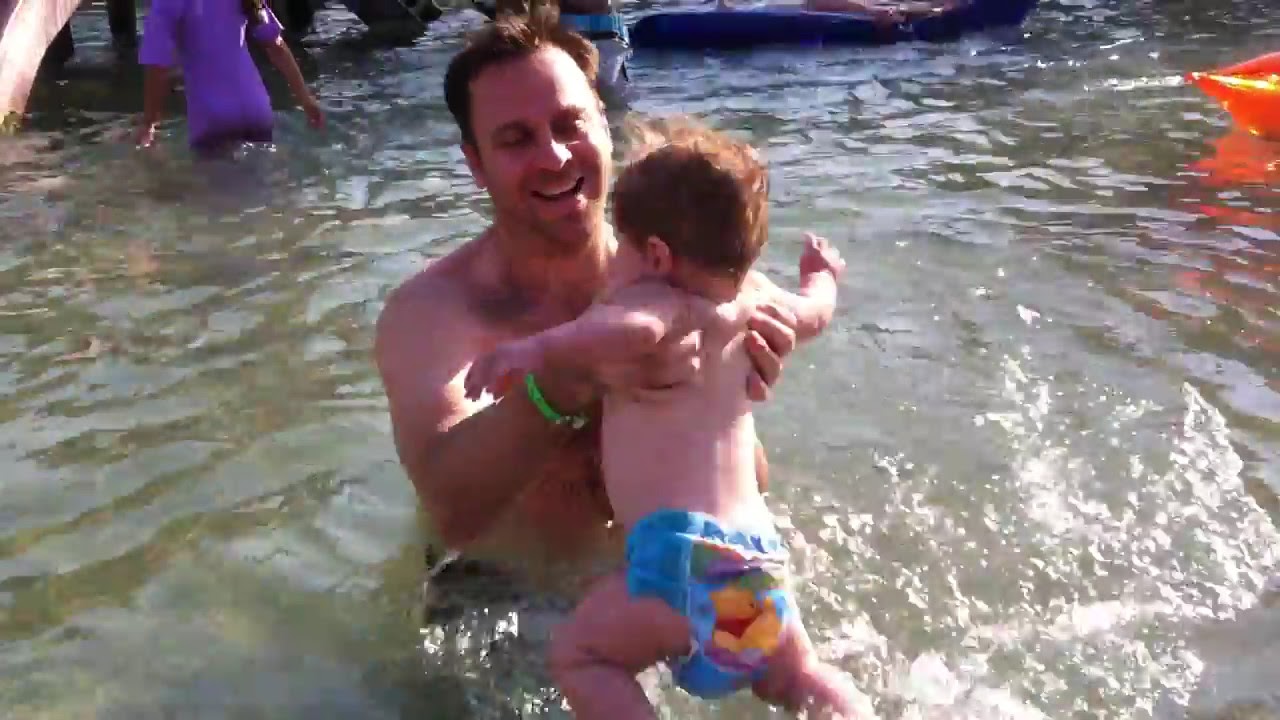A bright daytime photograph captures a joyful moment of a Caucasian man with short brown hair and a green bracelet on his right wrist, holding a baby in turquoise blue Winnie the Pooh-themed diaper in both arms. The man, who appears to be the child's father, is shirtless, revealing a furrier chest, and is smiling warmly at the baby who has orange hair and is raising its arms. Both are in a somewhat rippling greenish water, likely a lake or a lagoon. Nearby, an orangish boat is visible to the right, and a person in a purple shirt, seemingly a woman, walks away in the background. Other people and large rafts populate the scene, suggesting a lively water park or recreational area. The baby's back faces the camera while the man smiles at his child, creating a heartwarming atmosphere amidst the clear, sunlit water.